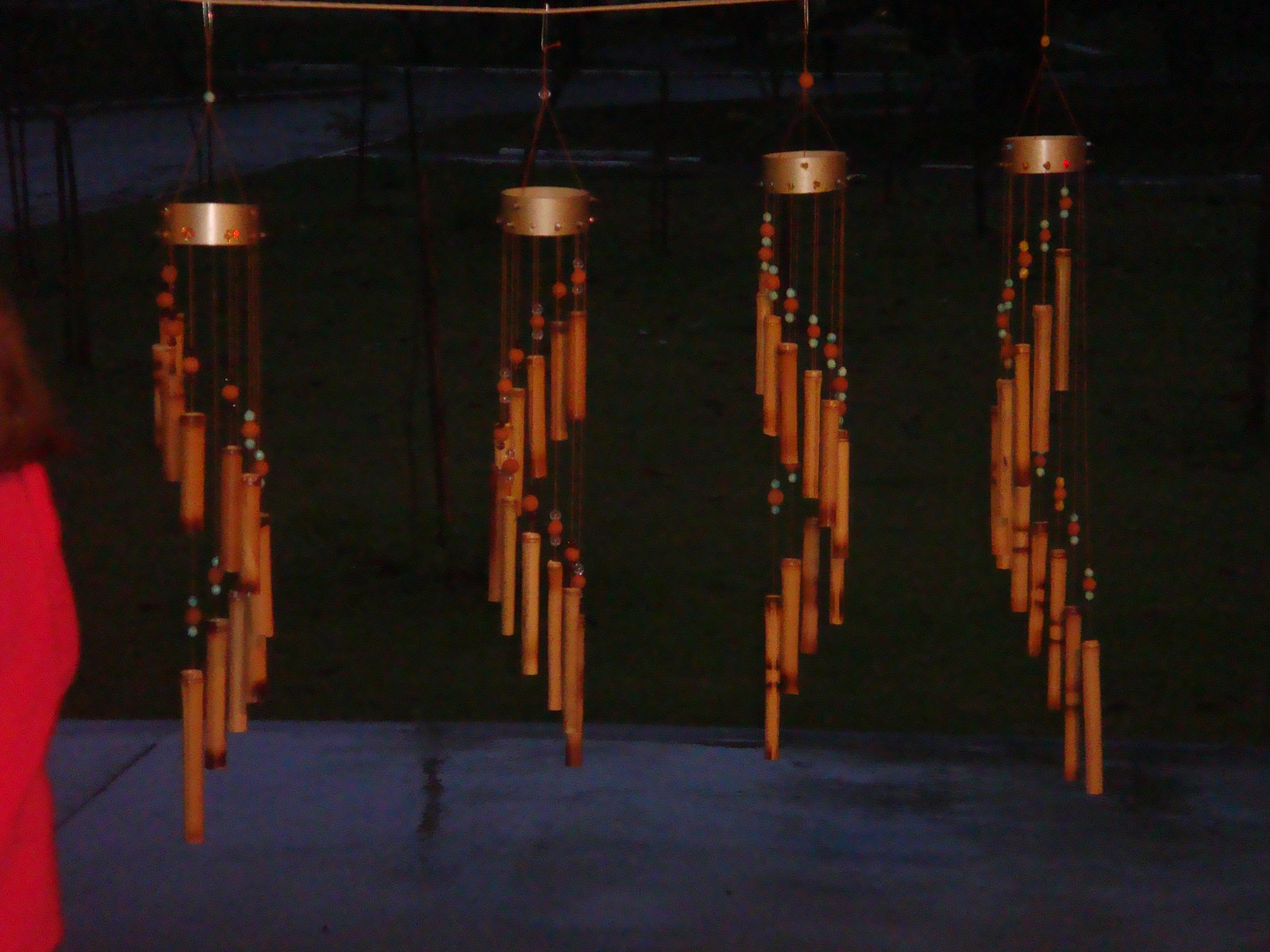In this nighttime photograph, taken in what seems to be a front yard or on a porch, four distinct wind chimes hang from a string. These chimes appear to be crafted from wood and adorned with colorful beads, predominantly featuring shades of red and light blue or turquoise. They are suspended from a central circular metallic ring embellished with reflective, red beaded designs. The chimes themselves have a brass-like appearance and are notably long. Off to the left edge of the image, the partially visible figure of a person with dark hair can be seen standing with their back to the camera, dressed in red. The dark background suggests a late hour, possibly around midnight, with the flash of the camera highlighting the intricate details of the wind chimes and the subtle reflections on the beads and metal.